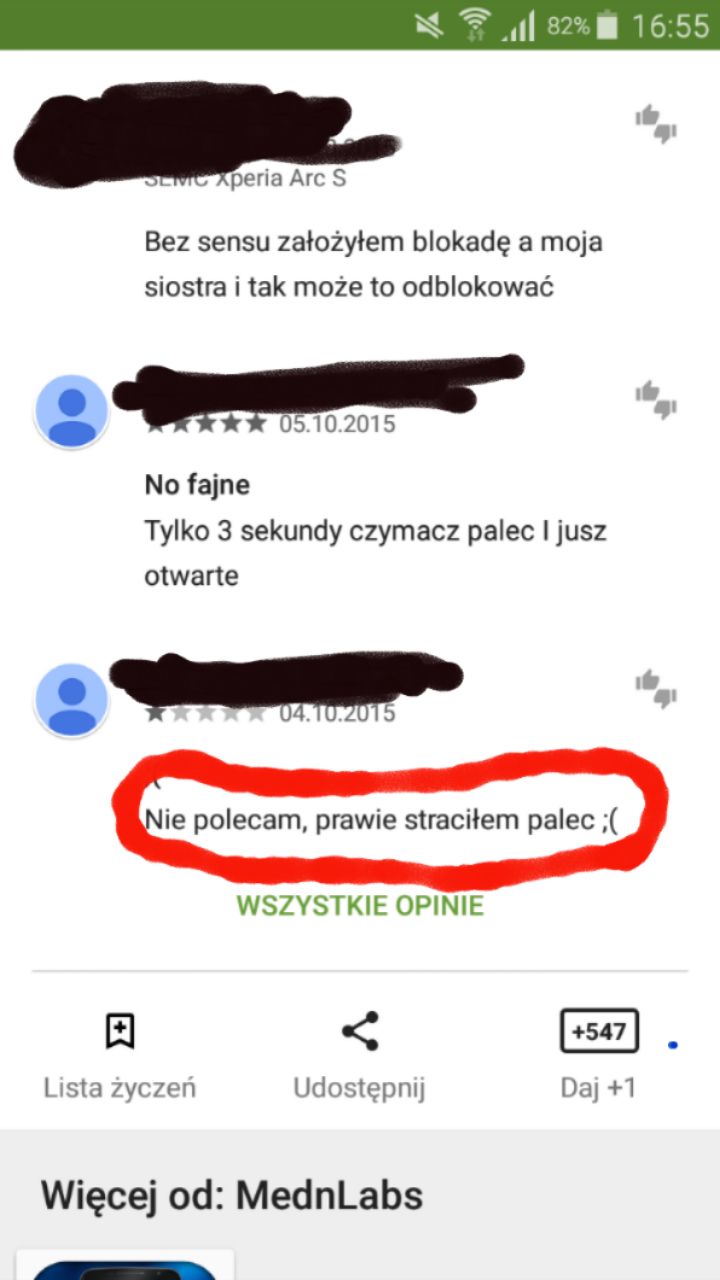This image is a vertical rectangular screenshot of a smartphone displaying a text chat written in Polish. The top of the screen features a dark green bar showing signal strength, time (16:55), mute icon, Wi-Fi strength, and battery life (82%). The names of the participants in the chat have been blacked out, resembling marks made with a black magic marker. One specific message, about four lines down, is circled prominently in red, highlighting the text that reads: "I set up a lock and my sister can unlock it anyway. Well, cool, just three seconds, finger and eat, open. I almost lost my finger," followed by a frown and a wink emoticon. Beneath this circled message, additional green text seems to provide more context regarding the highlighted post. At the bottom of the screen, there is more text in Polish along with a mention of "Medin Labs." There is also a section showing how many people are following the chat and how many liked it. This detailed screen grab captures a moment of frustration humorously shared via a text conversation.